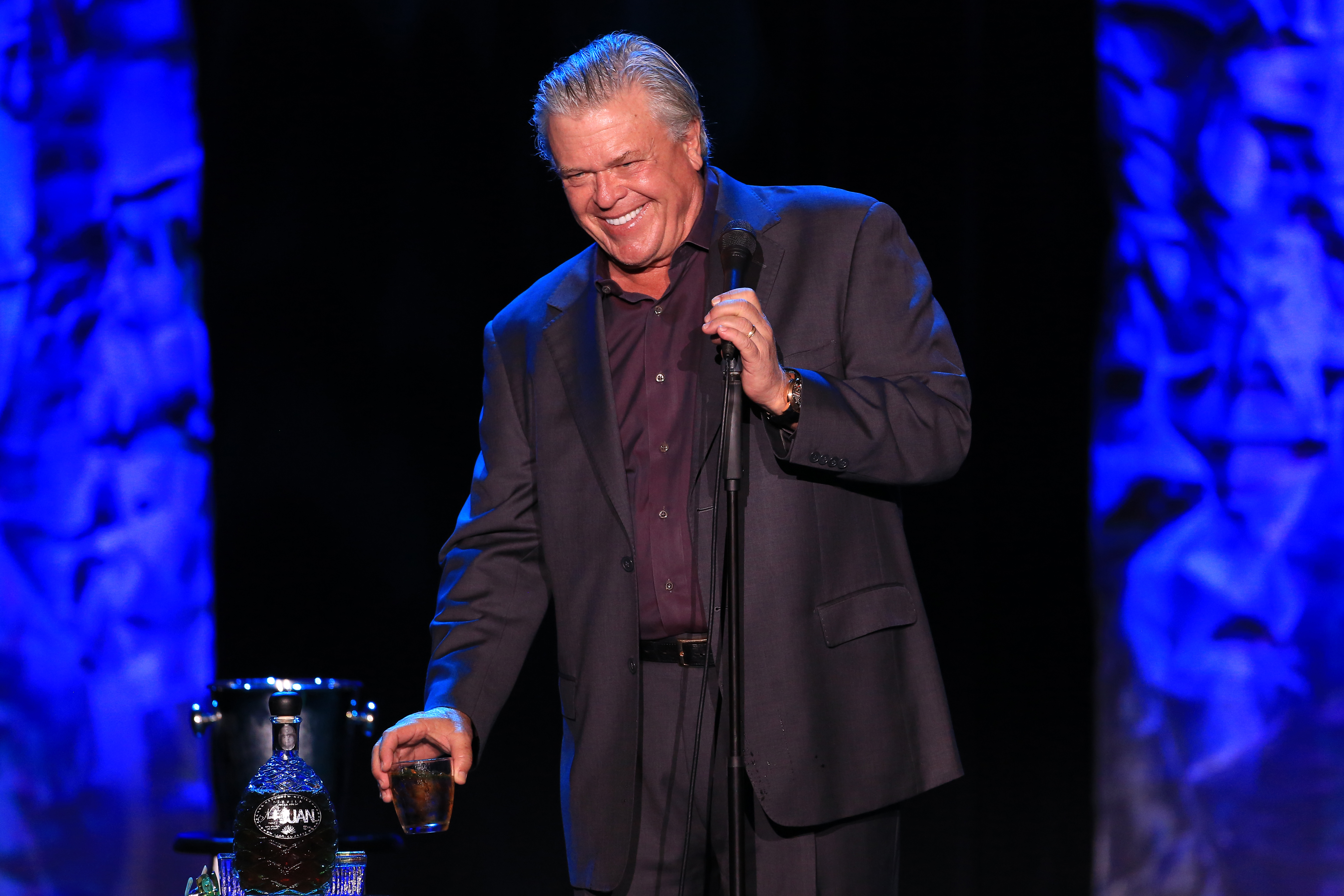The photograph captures an older white man, likely in his 60s or 70s, standing on a stage set against a black backdrop bordered by vibrant blue curtains on either side. He is dressed in black dress pants and a matching black dress coat with two undone buttons, revealing a silver-buckled black leather belt and a dark red, silk button-up shirt with the top two buttons left open. The man, who has gray, slightly balding hair and a heavier build, appears to be smiling and enjoying himself, possibly indicating he is a comedian. He holds a black microphone stand in his left hand, and his right hand grasps a small glass designed for drinking alcohol. Nearby, a table to his right holds a bottle of liqueur, adding to the ambiance of his performance.